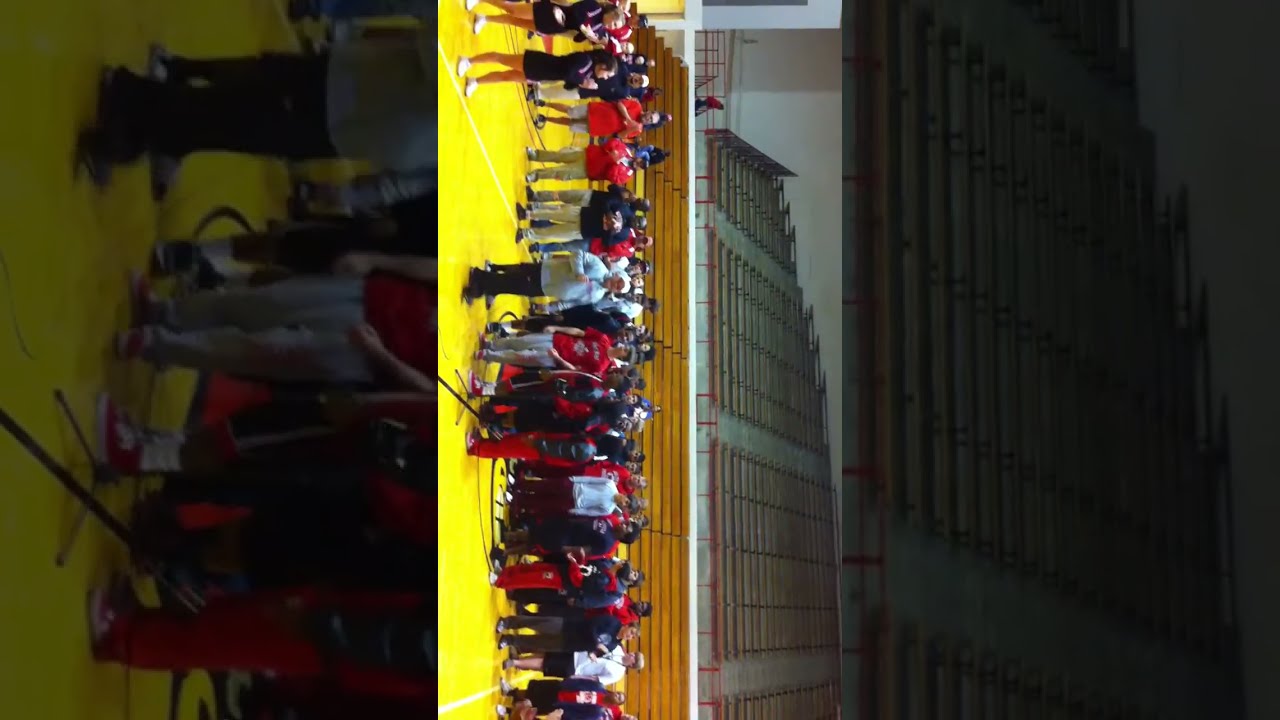This is a tilted portrait photograph capturing the interior of a sports arena, specifically a basketball court within a gymnasium. The image orientation is rotated 90 degrees clockwise, with large black bars filling the space on either side. A large group of mostly young black men, along with some white individuals, are gathered densely on the basketball court, many of them adorned in red jerseys and pants. One noticeable individual in the front left is an older white man wearing a white baseball cap and blue shirt, holding a microphone. Behind this assembly are pullout bleachers for spectators, with a dark surface visible above and possibly the bottom of a blue banner or windows at the top right (due to the rotated view), enhancing the setting's athletic ambiance.